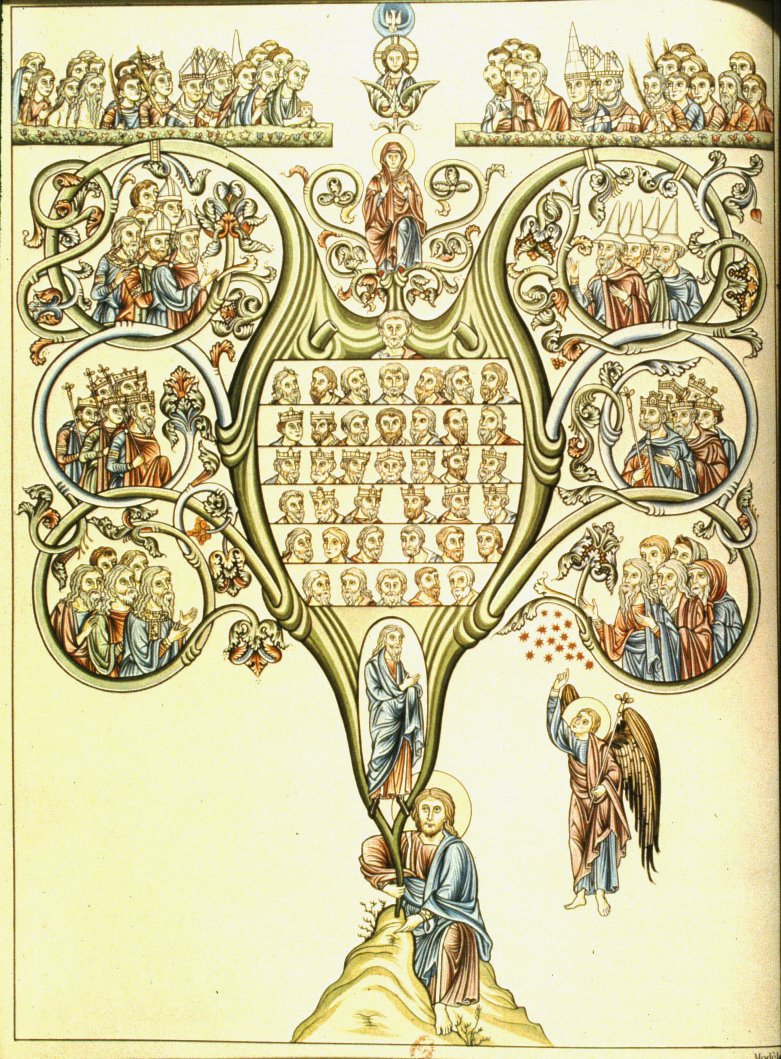The image is a highly detailed and vivid illustration resembling a family tree, primarily using shades of yellow, blue, and red. At the base of the tree, a figure that resembles Jesus Christ, dressed in blue and yellow, is holding up the trunk while seated on a rock or a hill. Branching out symmetrically from this central trunk, the tree forms circling patterns that encapsulate numerous faces of men, likely numbering between 50 to 60, suggesting a lineage or a collection of religious figures, many identified by halos. 

The left and right extending branches form circles housing clusters of faces all looking towards the central image. At the crux of these branches, above the central figure, a female figure dressed in blue and red robes occupies a prominent position. Further upwards, two rows of figures situated on what appears to be shelf-like structures flank either side, leading up to an image of an angel at the very top. The intricate and densely populated design of this tree-like structure combined with the halos, religious attire, and arrangement strongly suggests a depiction of biblical or holy figures, embedded within a golden and silver design backdrop.